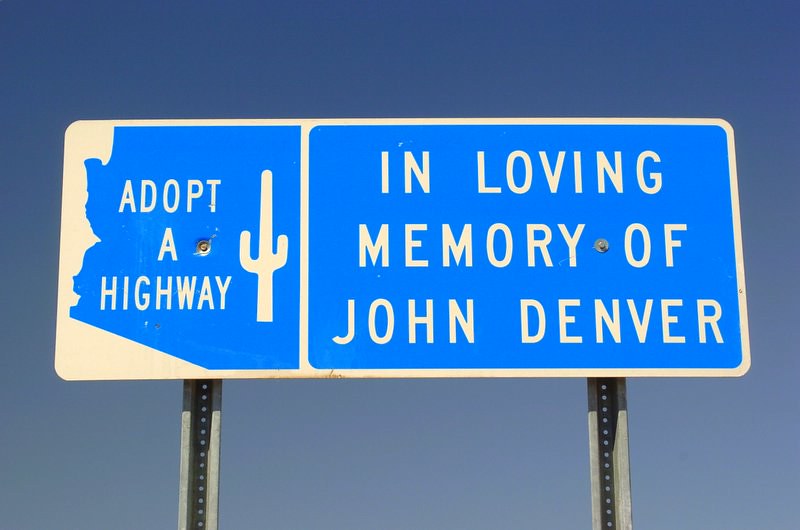This is a close-up, horizontal, color photograph of a slightly worn street sign against a cobalt blue sky that gradually fades to a lighter blue towards the bottom. The rectangular sign, which takes up the entire frame, is supported by two vertical gray metal poles, each featuring a line of serrated holes. The sign itself has a blue background with white lettering and a white rim along its edges. On the left side of the sign, underneath the outline of the state of Colorado, it reads "Adopt A Highway" above a white infographic of a cactus. The right side of the sign proclaims "In Loving Memory of John Denver" in bold, white block letters. Two visible screws attach the sign to the poles, with one screw positioned between the words "Memory" and "Of." A slight shadow is cast from the sign onto the poles, creating a subtle visual effect.